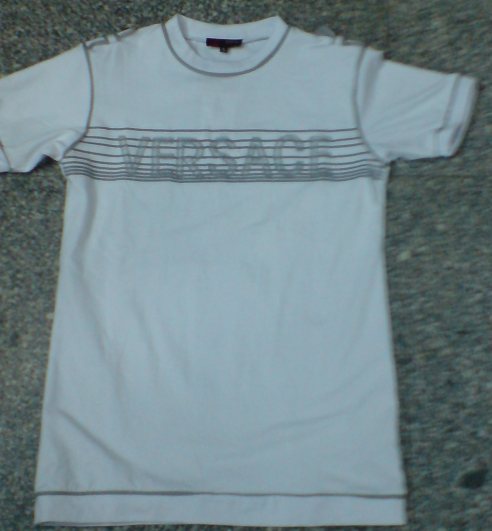This image features a white T-shirt displayed on a gray background. The T-shirt is adorned with meticulous gray stitching along the collar, sleeves, and hemline, adding subtle detail to its clean design. Prominently positioned on the front of the T-shirt is a bold block letter logo spelling out "Versace." The logo is overlaid with ten horizontal lines that vary in spacing, being more densely packed towards the bottom. The collar of the shirt includes a black rectangular tag, and just below it, there is a smaller square tag likely indicating the size of the garment.